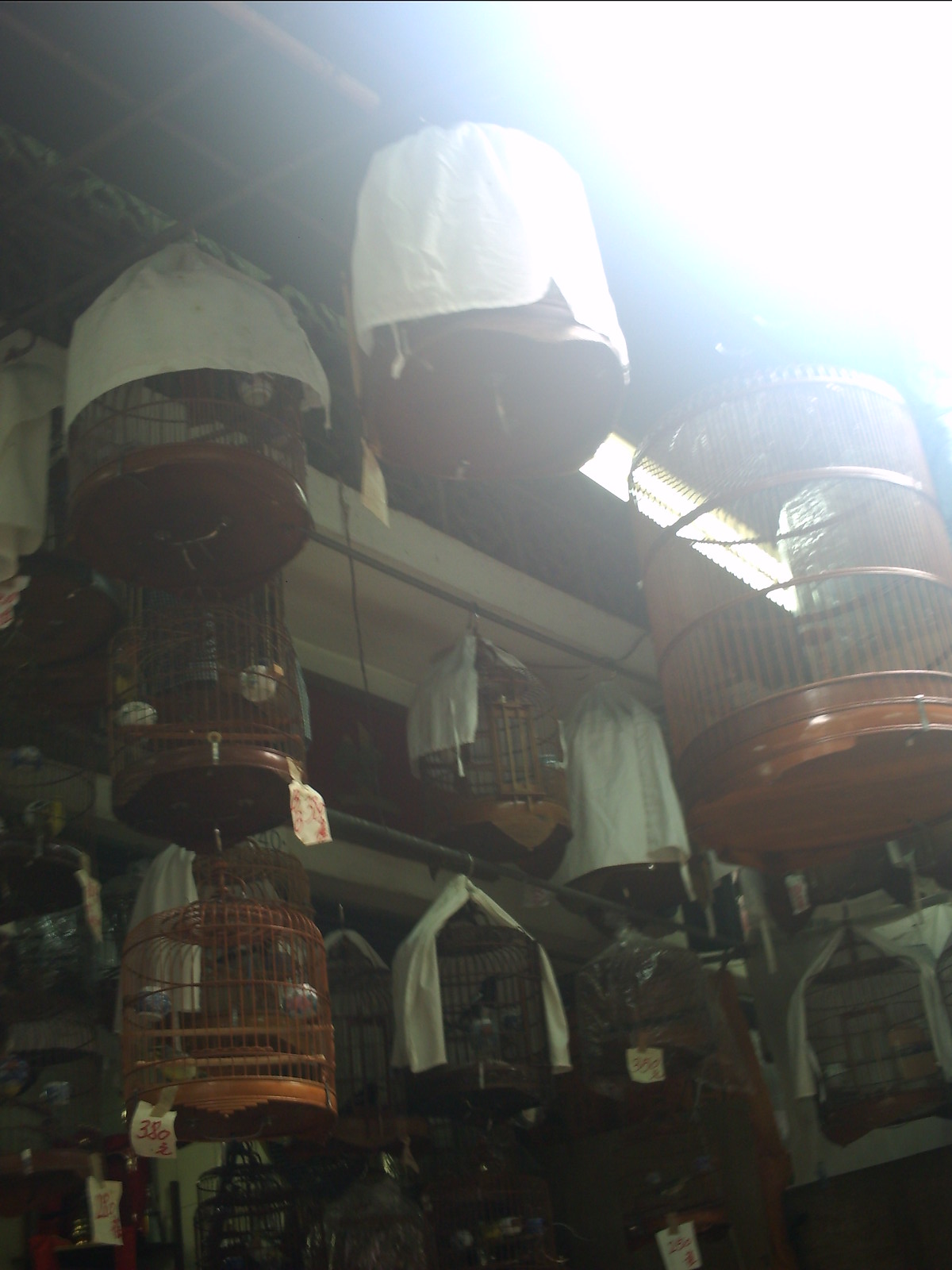This photograph captures a room densely populated with an array of bird cages, predominantly wooden or crafted from metal that mimics a wooden appearance. The cages adhere to a similar cylindrical or barrel shape, each fitted with a small hook for suspension from the ceiling or hanging rods that traverse the space at various levels. Seen from a floor perspective, the intricate bases and structural details of the cages are highlighted. 

Numerous cages, particularly those positioned in the top left and the background, are partially draped with white linen covers. The room is bathed in a bright light, emanating mainly from the upper right corner of the image, although the source—whether a window or artificial lighting—remains indistinct. This intense illumination saturates the upper right area with white light.

The scene is cluttered, filled overwhelmingly with bird cages that also line the walls on shelves. While perches and food bowls are visible within some cages, there are no birds present. Among the cages, the lower left one features a piece of white paper with red writing, indicating a price tag of 380 pounds. Overall, this detailed composition emphasizes the repetitive arrangement and the interplay of light and objects, creating a visually rich tapestry of bird cages.